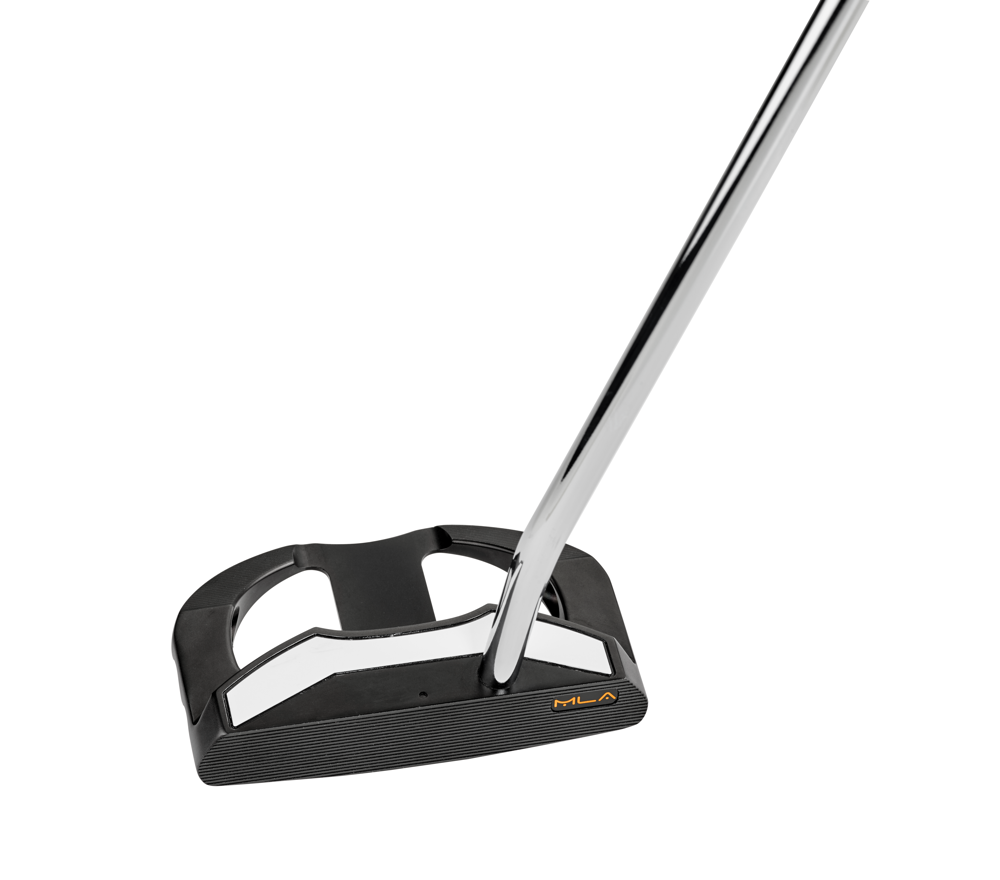The image depicts a highly engineered golf putter with a partially visible silver shaft, approximately eight inches in length, suggesting it is indeed part of a golf club. The putter's head is intricate, constructed from either black painted metal or plastic with a prominent white stripe on top. The head features a flat surface marked with the letters "MLA," accompanied by two open triangular sections and some grooves along the sides, hinting at unique design elements not commonly seen in traditional putters. The background is white, enhancing the focus on the putter's sophisticated and unusual appearance.